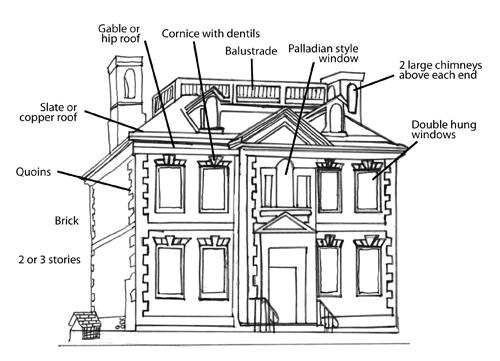This black-and-white diagram intricately details an early English-style two to three-story house. The house's exterior features are meticulously labeled: it boasts two substantial chimneys on each end and a slate or copper gable or hip roof adorned with a balustrade. The brickwork of the house is apparent, with the first and second floors each featuring four double-hung windows—two on either side of the centrally located front door. Above the entrance is a Palladian-style window, contributing to the house's classical aesthetic. A cornice with dentils lines the roof's edge, enhancing the architectural sophistication. The image's detailed annotations include smallish black font labels connected by lines to the respective architectural elements, offering a comprehensive schematic of the house's design components. A rail flanks each side of the doorway's entrance, although no stairs are visible.